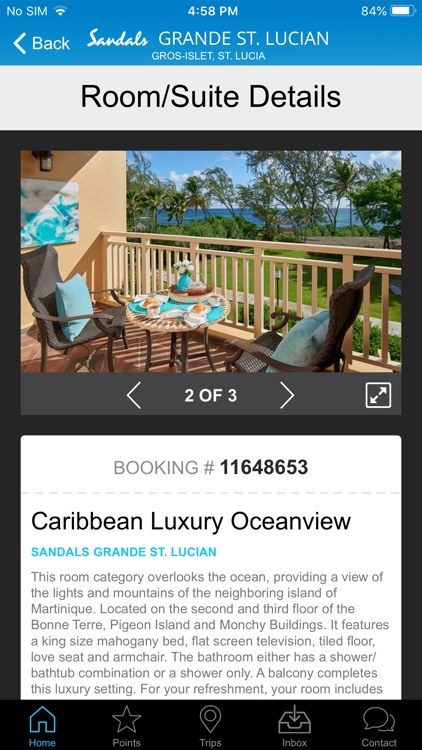This image showcases a social media-style post with a blue border at the top of the screen. In the upper left-hand corner, there's a white font displaying "No SIM" next to a Wi-Fi icon, and nearby, it shows the time as 4:58 p.m. and the battery life at 84%, indicated by a nearly full white battery icon.

Below this, a navigation bar features a back arrow next to the word "Back," followed by the text "Sandals Grand St. Lucien, Gross Islet, St. Lucia" and "Room/Suite Details." The central image depicts a cozy, brown and teal-colored patio set on a yellowish-hued balcony. This balcony overlooks a lush, green landscape leading to a distant view of blue water.

The post provides a booking number "11648653" for a Caribbean Luxury Ocean View stay at Sandals Grand St. Lucien. The room category benefits from an ocean view, offering a sight of the illuminated mountains of the neighboring island of Martinique. Located on the second and third floors of the Monterey, Pigeon Island, and Monshea buildings, this accommodation features a king-size mahogany bed, a flat-screen television, tiled flooring, a loveseat, and an armchair. The bathroom is equipped with either a shower-bath combo or a standalone shower. Additionally, a balcony completes this luxurious setting.

At the bottom of the screen, the navigation menu includes options for "Home," "Points," "Trips," "Inbox," and "Contact." The text cuts off after listing some room amenities, leaving details unfinished.